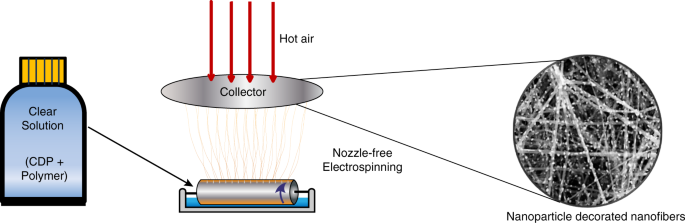The image is a flowchart-style scientific diagram set against a white background. On the left-hand side, there is a digital illustration of a blue bottle with an orange screw-on cap. The bottle is labeled "Clear Solution CDP plus Polymer." An arrow points diagonally downward from the bottle to a silver cylinder, attached to a rod between two posts. The diagram is titled "Nozzle-Free Electrospinning." Pink waves ascend from the cylinder to a silver disc, labeled "Collector." Four red arrows labeled "Hot Air" point downward toward the collector. To the right, two lines extend from the collector to a circle on the right edge of the diagram. This circle is labeled "Nanoparticle Decorated Nanofibers" and features white fibers against a black background, depicting the final product of the process.